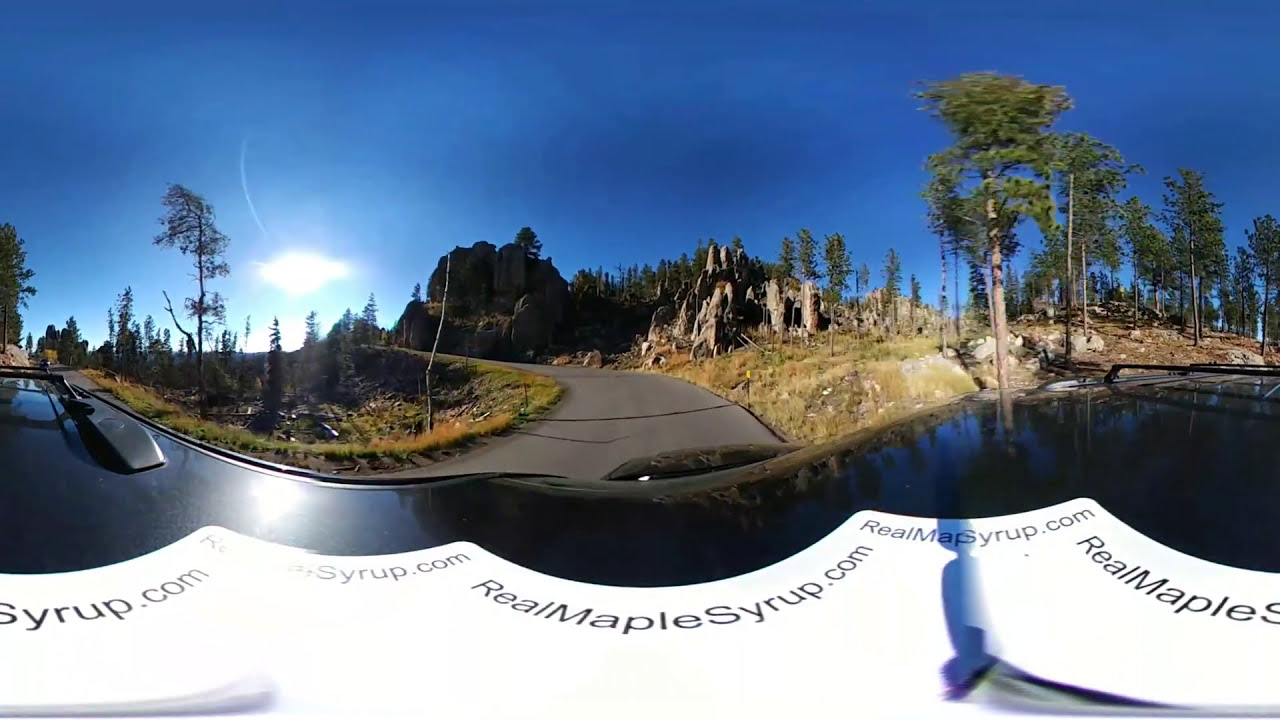The image captures a outdoor scene from the perspective of someone inside a vehicle, with the top of the hood visible in the foreground. A sticker on the hood repeatedly displays the text "RealMapleSyrup.com." At the bottom of the image, there's a wide white section also featuring the same website text. The central focus is a winding path or road that stretches out from the bottom toward the horizon, flanked by green grassland and scattered trees. The trees nearer to the far end of the path appear larger and darker green. Among the trees and grass, there are some rock formations, adding texture to the landscape. The sky above is a mix of various shades of blue, with a notable white sun situated towards the left side, casting a bright light over the scene.